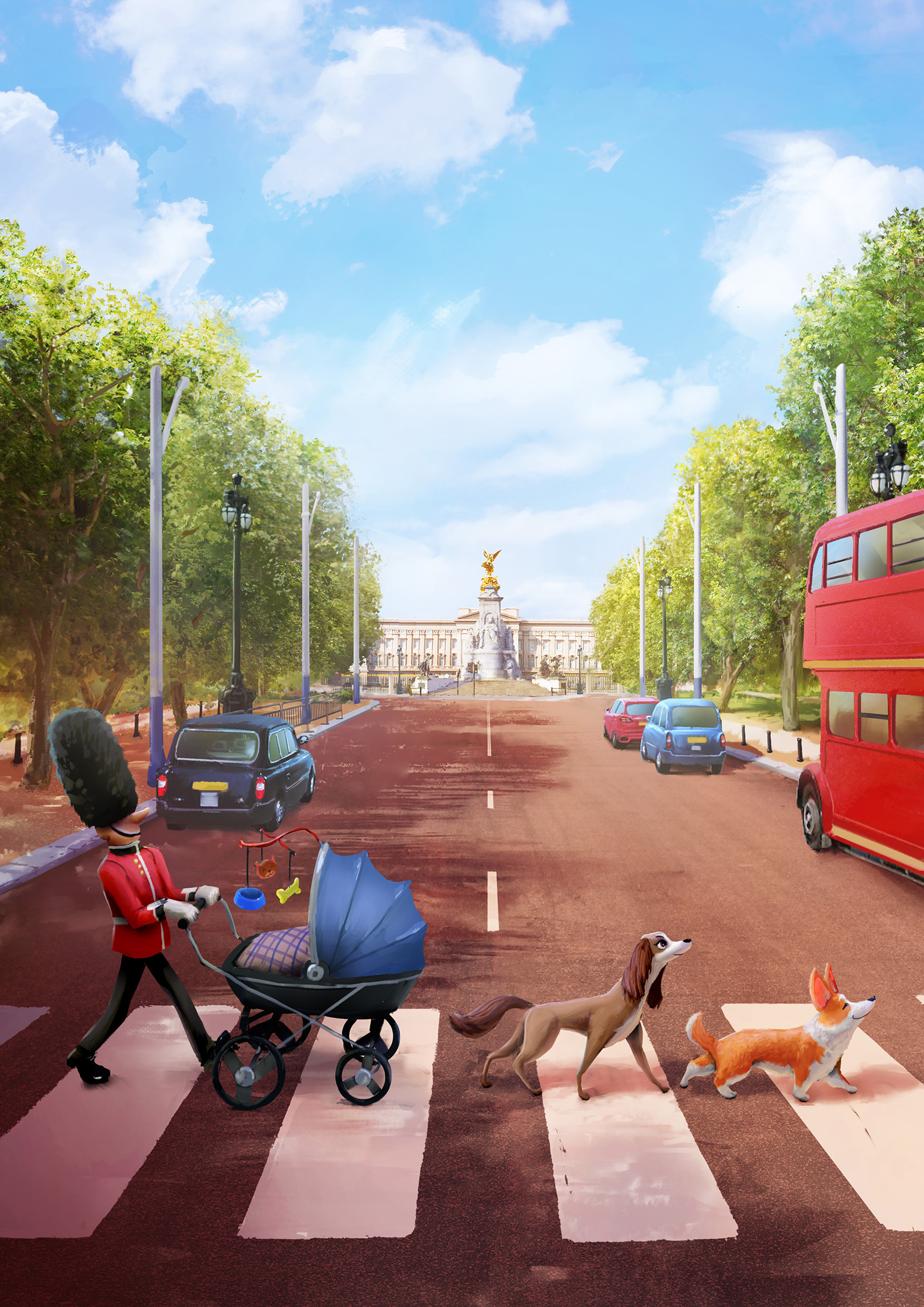The image is a detailed digital cartoon illustration depicting a classic British street scene. At the center, a traditional British Guardsman, easily recognized by his tall black busby, red coat with white patterns, black trousers, and boots, is pushing a blue baby stroller. The stroller features a top awning, a wind mobile hanging above, and a baby wrapped in a checkered blanket inside. Two dogs precede the stroller on a zebra crossing: a brown spaniel with long, down-facing ears, a fluffy tail, and a mix of orange and dark brown hair on its ears, and an orange and white corgi with pointy ears and a short tail. The background reveals a bustling British setting with a black sedan, a blue car, a red car, and a distinctive red double-decker bus. The scene is framed by green trees, silver street lamps, and hints of a white colonial building, enhancing the charming and quintessentially British atmosphere of the illustration.